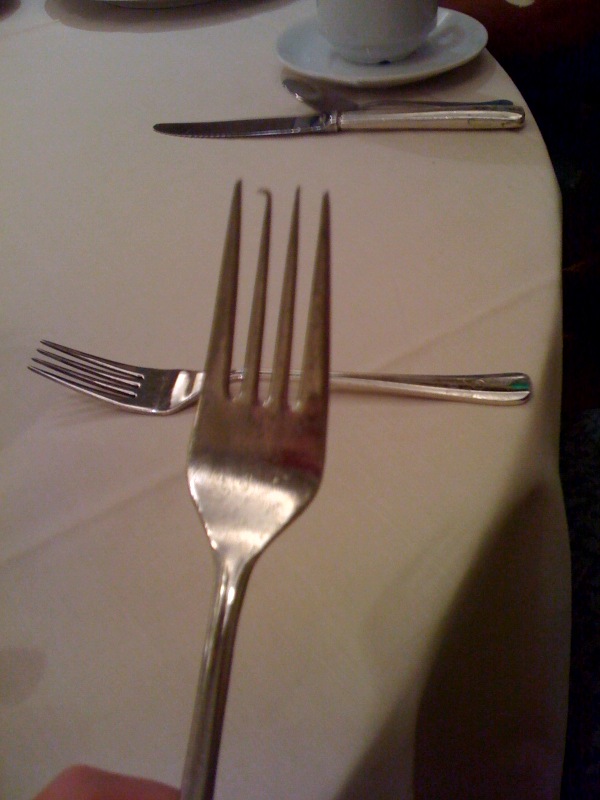This indoor color photograph features a close-up of a hand holding a used silver fork vertically, tongs pointing upward, with a noticeable bend on the second tine from the left. The background reveals a white-linen-covered round table, partially visible, taking up the majority of the frame. On the table, horizontally laid, is another fork, a butter knife, and a spoon, all in a typical table setting position. To the right, partially out of frame, is a white china teacup on its saucer. The photograph shows a stark contrast between the focused objects and the slightly out-of-focus hand holding the damaged fork prominently in the foreground, capturing a moment likely of interest due to the fork's bent tine. The setting implies either preparation for or the aftermath of a meal.